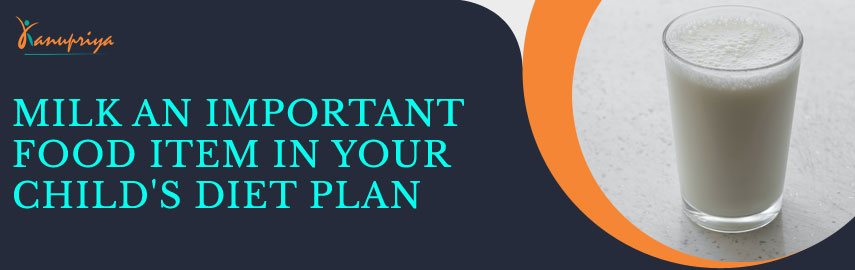The advertisement features a horizontally oriented design with a prominent black background accented by a navy-blue section and vibrant turquoise text. The main text in uppercase reads, "MILK, AN IMPORTANT FOOD ITEM IN YOUR CHILD'S DIET PLAN," displayed in a mint-green hue against the dark backdrop. On the left side, there is an indistinct logo or brand name in the upper left corner, possibly reading something akin to "Priya," highlighted in gold writing that is partially obscured. 

To the right of the text, the layout includes a graphical element—a looping orange line that transitions into a larger circular frame encompassing a full glass of milk, perched on what appears to be a countertop surface. The glass of milk is depicted with a slight foam at the brim, emphasizing its freshness. The entire poster's layout is horizontal, creating a rectangular shape that neatly balances the textual and visual elements.